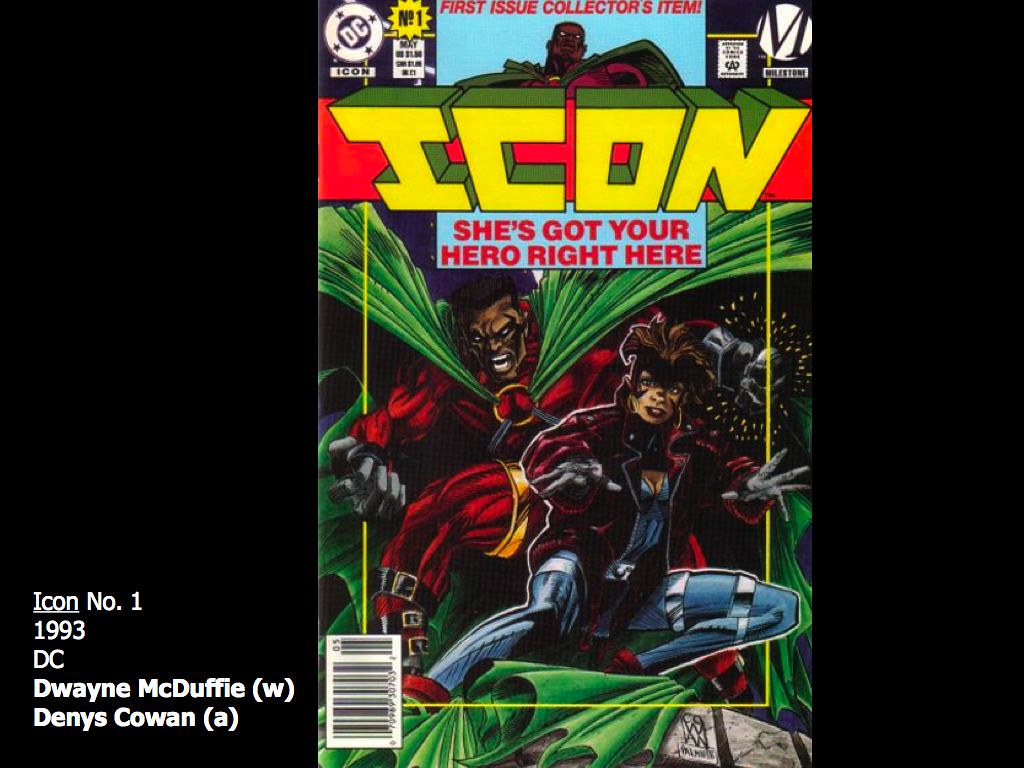This is a detailed description of the cover of a DC comic book, specifically the first issue of "Icon," published in 1993. Prominently displayed in the top left corner is the DC logo, signifying its publisher. At the very top, bold text announces this as a "first issue collector's item." The title "Icon" is emblazoned in large, block yellow letters. Below the title, the phrase "she's got your hero right here" is inscribed. The central image features two African American superheroes. The woman on the right, with short hair, is donned in a long, heavy leather jacket and gloves. The man posing next to her is dressed in a skin-tight red suit coupled with a large green cape. The left and right borders of the cover are black, with the bottom left corner containing a crucial informational snippet in white text: "Icon, number one, 1993, D.C., Dwayne McDuffie, writer, Denys Cowan, artist." This text also clarifies the creators' roles, with W standing for writer and A for artist.